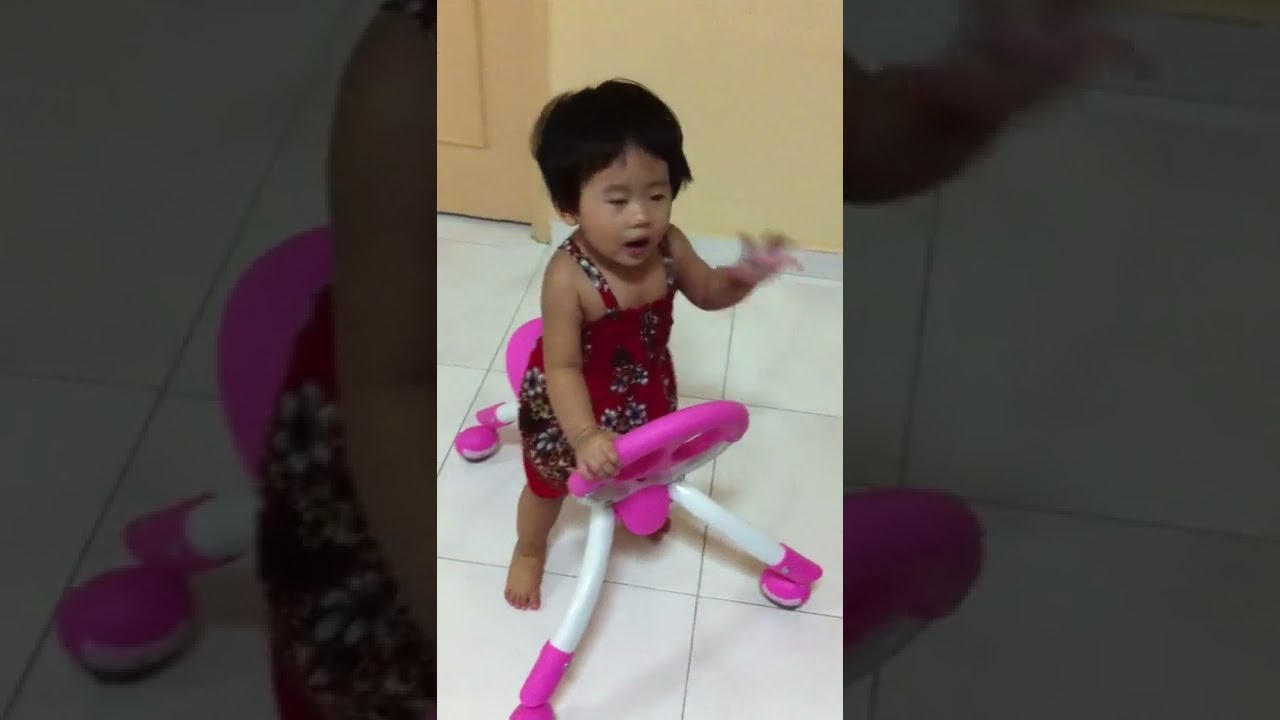The horizontal rectangular image, which is somewhat blurry and has wide black borders on both sides, captures a scene primarily in the center of the frame. At the center stands a little girl, seemingly around two years old, with short black hair styled in a bowl cut. She is dressed in a sleeveless red dress adorned with black and white floral patterns. The child is straddling a toy with long white arms and legs, which sport purple boots and mittens. This toy supports her weight as she stands on it. The girl and the toy are positioned on a white tiled floor composed of square tiles. The room's walls are a pale beige or yellowish-apricot color, accented with white baseboards. In the upper left corner, the bottom part of a brown door is visible, adding context to the indoor setting.